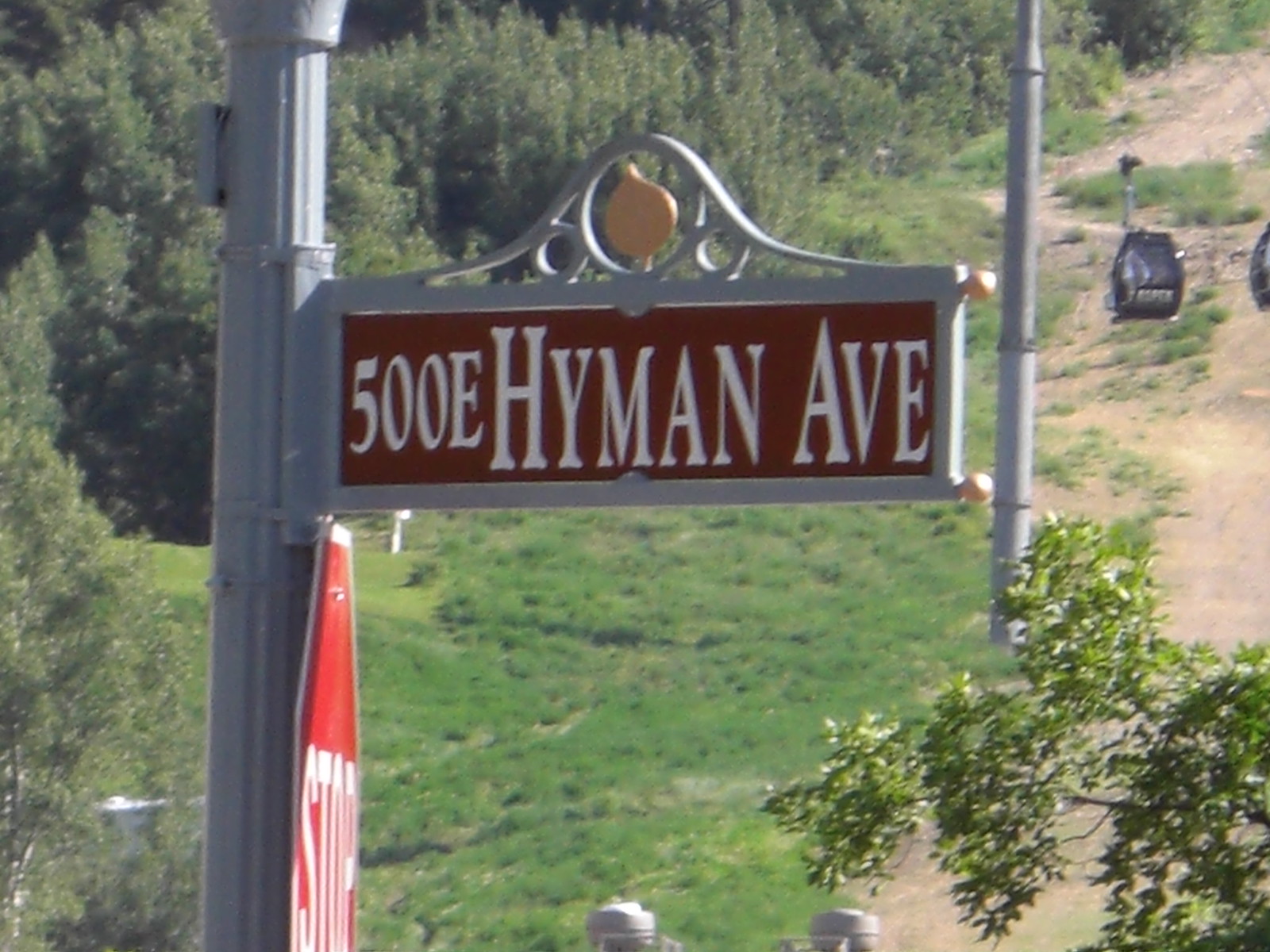This photograph captures a large, ornate street sign mounted high on a robust metal pole. Directly beneath it, a red stop sign is affixed, facing the opposite direction. The street sign, framed in metal with an elegantly curved top, is a rich chocolate brown color and displays the text "500 East Hyman Avenue" in white letters. In the background, a green grassy hill is visible, featuring a dirt entrance where a couple of cars are parked. Beyond this area, a trailhead begins, leading into a densely wooded area.